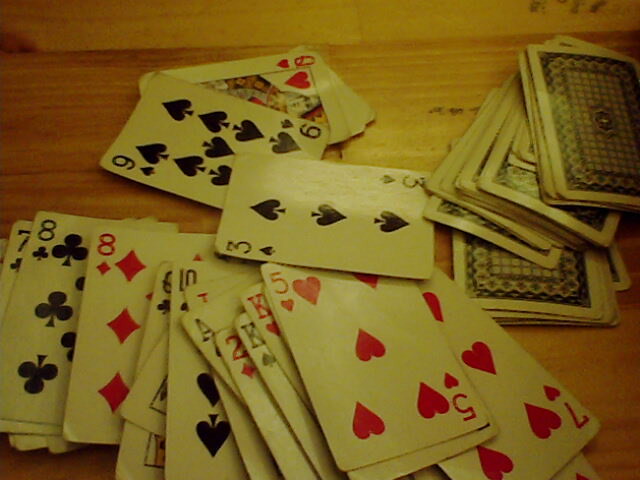The image features a wooden table as the background, extending from the top to the bottom of the frame. The table exhibits a variety of brown shades, with the top left corner having darker wooden markings, while the top right and bottom right corners display lighter brown tones.

Scattered across the table are numerous playing cards. In the right middle section of the image, several cards are flipped face down, revealing their intricate back design. The back features a large, vertically-oriented black rectangle with multiple tiny squares within it, centered around a hexagon-shaped logo.

In contrast, the bottom left of the image shows cards lying face up. Notably, the Queen of Hearts, Nine of Spades, and Three of Spades are visible in the middle of the image. The bottom half of the image also displays other face-up cards, such as the Five of Hearts, Seven of Hearts, and King of Hearts. Additionally, the bottom left corner reveals the Eight of Diamonds and Eight of Clubs stacked on top of each other, with all face-up cards forming a cluttered, layered arrangement.